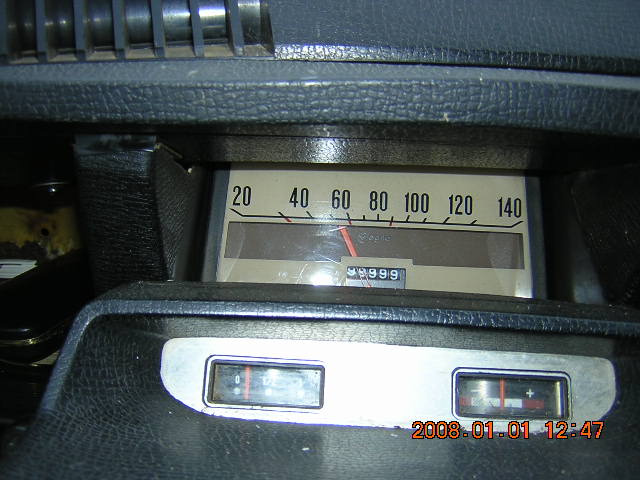In this close-up image, we observe what appears to be an old-fashioned car dashboard. Dominating the center is an antique dial featuring a speedometer, indicated by the range of 20 to 140, though the units are unspecified. The numerals and their somewhat faded dark yellow hue give the dial a vintage feel, characteristic of older vehicles. Below the speedometer's display, there is a set of numbers "99999," reminiscent of a mechanical odometer or a locker combination lock. Additionally, a date "2008-01-01" and a time "12:47" are visible, suggesting the presence of a digital display integrated into the dashboard. The upper section of the image includes what seems to be dashboard leather, reinforcing the impression that this is indeed part of a car’s interior. The background is cluttered with indistinguishable objects, adding to the antique and slightly cryptic ambiance of the scene.